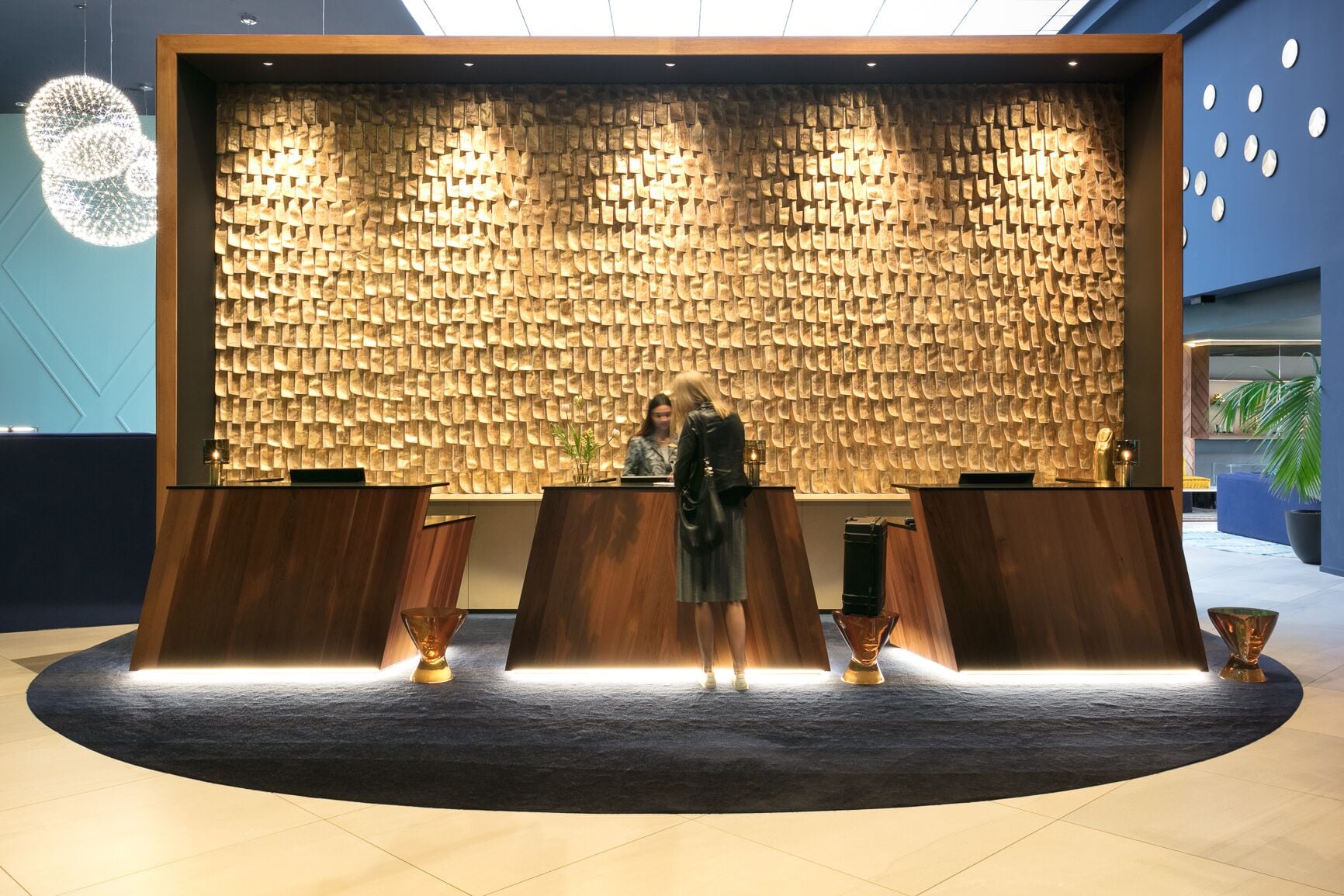The photo captures a check-in area resembling that of a museum or possibly a science or history institution. The area features three wooden reception counters, all situated on a large deep gray circular rug. There are two women at the central counter—one is a receptionist working behind a computer, and the other is a guest standing with her back to the camera. The backdrop behind the reception area includes a prominent golden rectangular structure, approximately 15 to 20 feet high, with cascading lights, adding a dramatic flair to the setting. The walls in the background are a deep blue, adorned with what appear to be silver transparent balls hanging from the ceiling, contributing to the modern and striking decor.